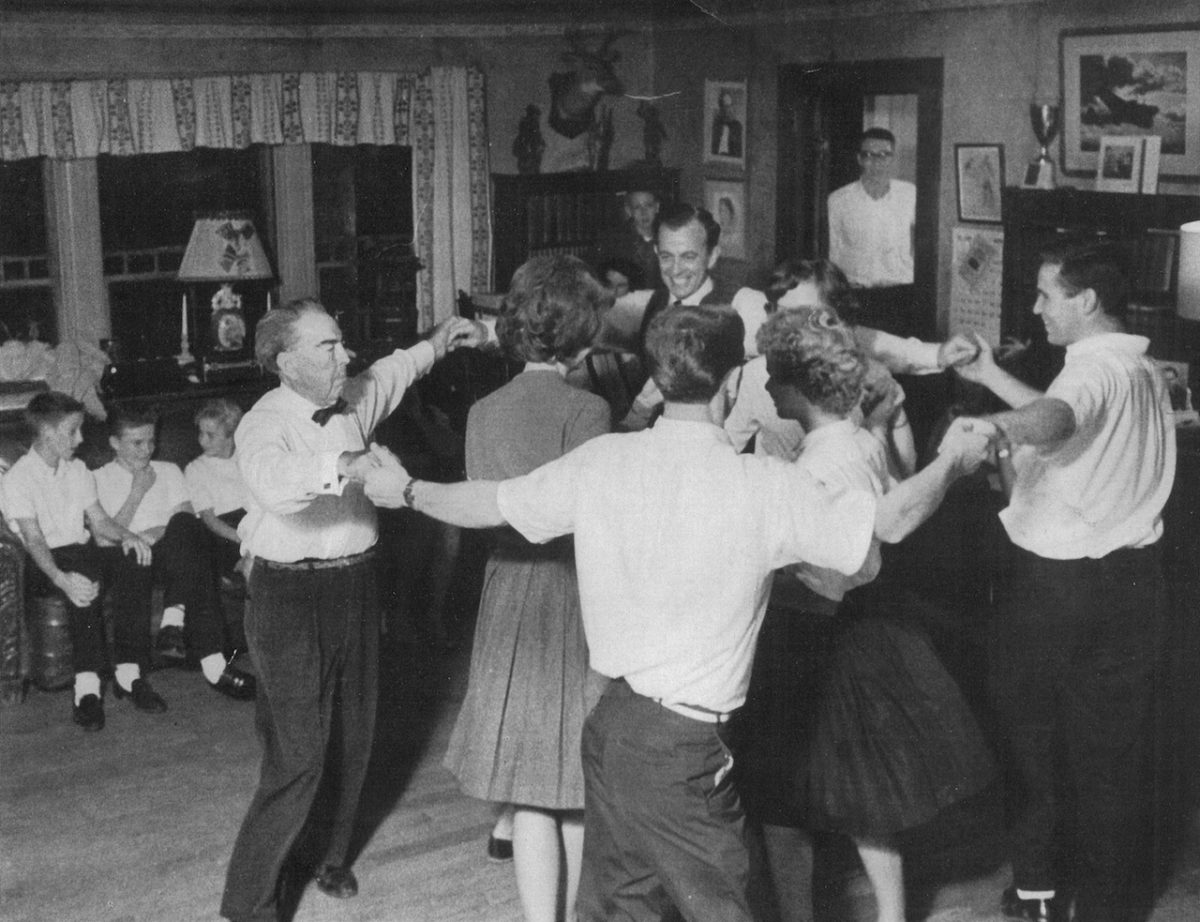This black and white photograph, likely taken in the 1950s or 1960s, captures a joyous scene in a large living room during a lively gathering. The room is decorated with various items, including pictures on the walls, a bookshelf, cupboards, lamps, and patterned curtains on a large window. A shelf adorned with trophies and a mounted deer head is also visible. In the foreground, a group of four men, all dressed in white shirts—some with long sleeves, some with short sleeves, and one even wearing a vest and bow tie—hold hands in a circle and dance around three women in skirts or dresses. The men’s expressions vary from neutral to smiling, conveying the festive atmosphere. On the left-hand side of the image, three boys, all wearing black pants and white shirts, sit on a couch, laughing and enjoying the scene. Behind them, a lamp and a large curtained window can be seen. In the background, a man with glasses, observing the fun, stands in a doorway. The wooden floor of the living room adds warmth to the vibrant energy of people dancing and engaging with one another.